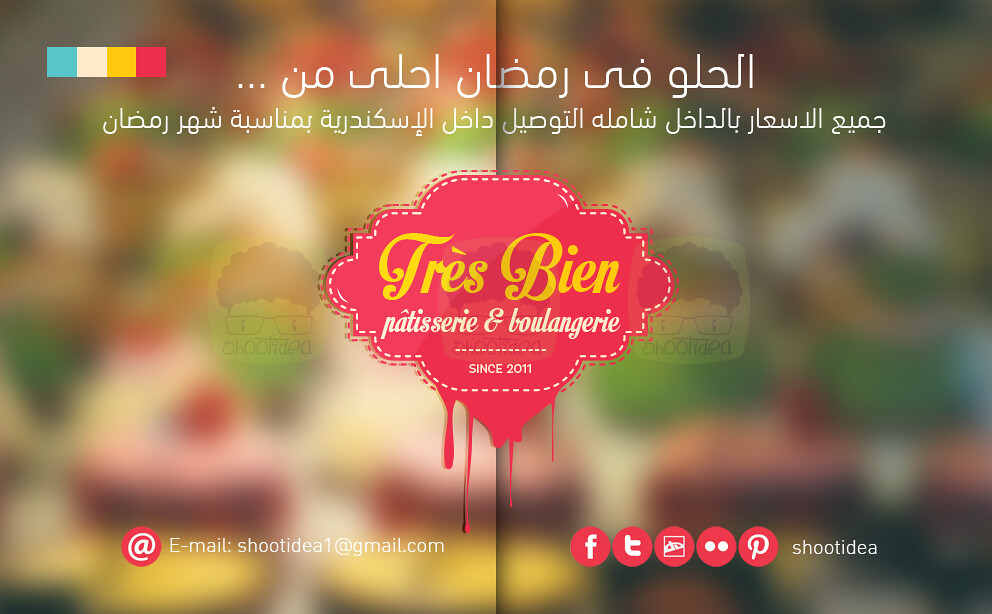The image, which has a rectangular shape, is an advertisement for an establishment named Très Bien Patisserie and Boulangerie. The background is blurred, with abstract splashes of various colors, resembling sweets or cupcakes. At the top left corner, there is a bar divided into four colored sections: turquoise, white, yellow, and pink. Above this bar, there is text in an unfamiliar language, possibly Hebrew or Arabic, written in white.

Dominating the center of the image is a hot pink logo that looks like a dripping ice cream scoop. Inside this logo, "Très Bien" is written in yellow, with "Patisserie and Boulangerie" below it in white. Below this text, there is a mention of "Since 2011," indicating the establishment's founding year.

Towards the bottom of the image, the email address shootidea1@gmail.com is prominently displayed in white. Additionally, icons for social media platforms such as Facebook, Twitter, and Pinterest are lined up on the bottom right, along with the text "shoot idea." The overall design suggests a vibrant and inviting atmosphere aimed at promoting the patisserie and boulangerie.